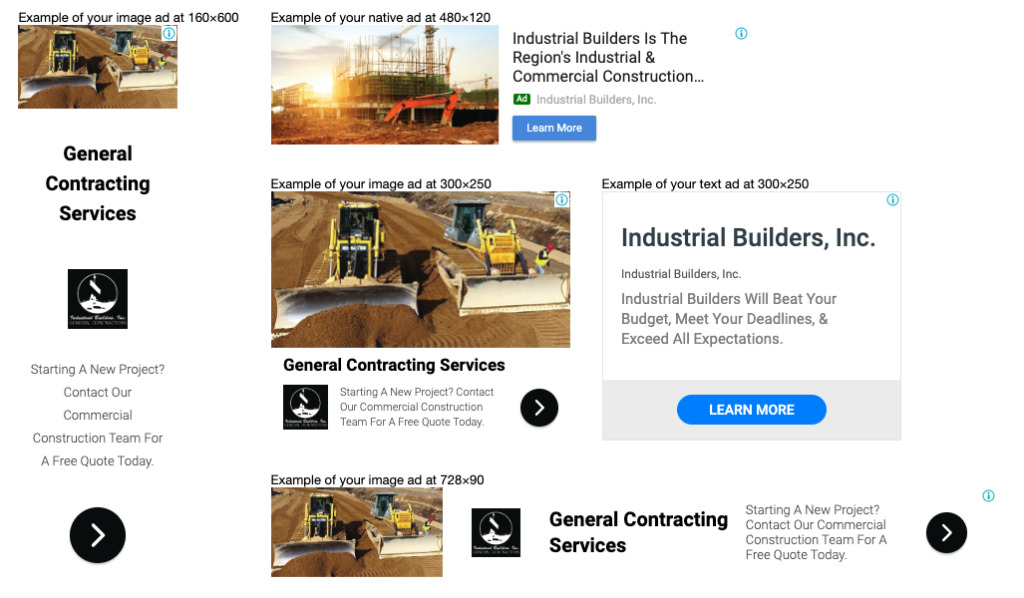The image depicts a well-designed promotional material for a general contracting company. The layout resembles a trifold brochure, meticulously arranged in three distinct panels as if shown in a print-ready PDF format but displayed flat on a digital screen. 

On the left panel, the title "General Contracting Services" stands out prominently. Below the title, there are several small, strategically placed images featuring heavy machinery such as backhoe loaders, forklifts, and cranes, emphasizing the company’s robust capabilities in handling large-scale projects. 

The center and right panels contain marketing copy under subtitles like "Industrial Builders in the Region" and "Industrial and Commercial Construction." Additionally, a variety of small icons are dispersed throughout the brochure, complementing the textual content and adding a visual hierarchy to the information. 

The brochure balances text and visuals effectively, creating an engaging and informative overview of the general contracting services offered by the company.